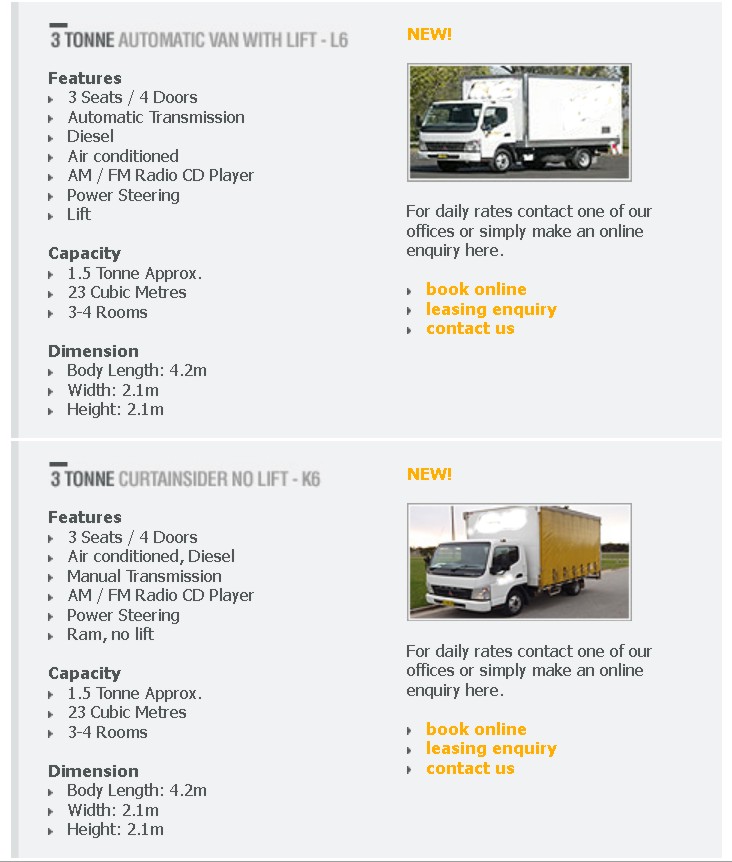This screenshot captures a webpage listing two delivery vans available for sale. The exact website name is not provided. At the top right, there is an advertisement for a white delivery van, labeled as 'New'. The accompanying text reads, "For daily rates, contact one of our offices or simply make an online inquiry here. Book online, leasing inquiry, contact us." Detailed specifications for this van include: 

- Model: Three-ton automatic van with lift, L6 
- Features: Three seats, four doors, automatic transmission, diesel engine, air conditioning, AM/FM radio with CD player, power steering, and a lift 
- Capacity: Approximately 1.5 tons, with a volume of 23 cubic meters, suitable for three to four rooms 
- Dimensions: 4.2 meters in length, 2.1 meters in width, and 2.1 meters in height 

Below, there is another advertisement on the right side for a different delivery van, also labeled 'New'. This van features a dual-color scheme with an orange side and a white front cab. The text beneath reads, "For daily rates, contact one of our offices or simply make an online inquiry here. Book online, leasing inquiry, contact us." Specifications for this van are:

- Model: Three-ton curtain slider, no lift, K6 
- Features: Three seats, four doors, manual transmission, diesel engine, air conditioning, AM/FM radio with CD player 
- Capacity: Approximately 1.5 tons, with a volume of 23 cubic meters, suitable for three to four rooms
- Dimensions: 4.2 meters in length, 2.1 meters in width, and 2.1 meters in height